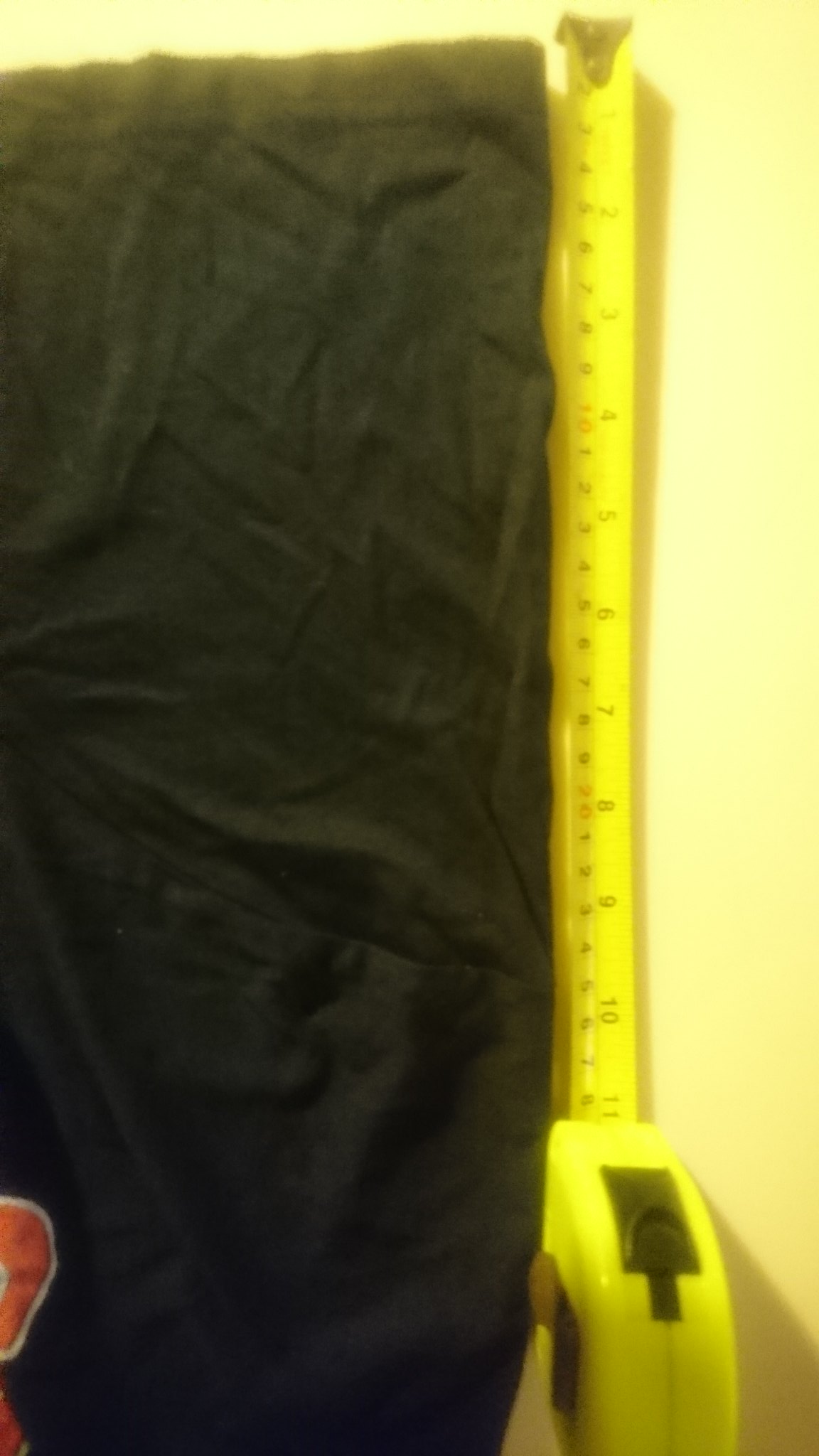A bright yellow measuring tape with clear black numbers spans across a wrinkled black cotton t-shirt, capturing a partial measurement of 11 inches. The tape extends from the end of the shirt at the top of the image towards the bottom, positioned on a yellow-cream colored tabletop. A subtle detail of the shirt includes a small spot of red writing located in the bottom left corner of the garment. The measuring tape does not cover the entire length of the shirt, stopping approximately two-thirds of the way up due to the framing of the photograph.